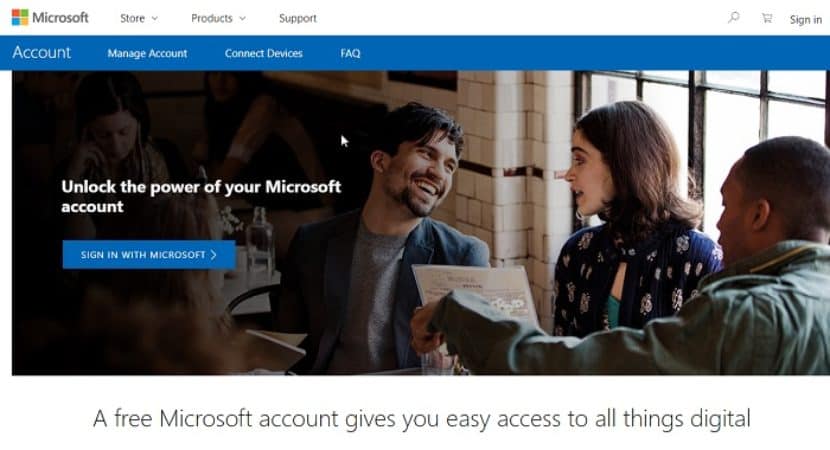Caption: 

"Unlock the power of your Microsoft account: Sign in with Microsoft to gain seamless access to all digital services. In this vibrant stock photo, three young, trendy individuals are seen enjoying their time at a cozy coffee shop in a bustling downtown area. They’re seated at a wooden table, engaged in animated conversation and laughter. The diverse group features a white man, a white woman, and a Black man who is casually reading the menu. Above them, the Microsoft webpage is displayed with a straightforward layout, featuring a white navigation bar at the top with options for 'Store,' 'Products,' 'Support,' a search icon, 'Sign in,' and 'Cart.' Below, a blue navigation bar offers links to 'Account,' 'Manage Account,' 'Connect Devices,' and 'FAQ.' The atmosphere is relaxed, reflecting the ease and simplicity of managing a Microsoft account."